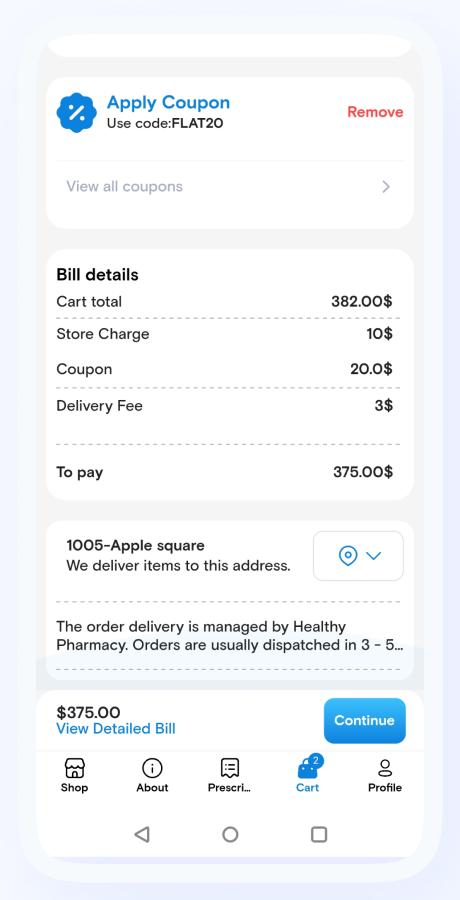This image showcases a detailed invoice layout. At the top left corner, there is a white box labeled "Apply Coupon" in bold blue text. Directly below this, it instructs "Use code: FLAT20" with a blue circular badge to its left, featuring a white percent symbol in the center. To the right of this section, there's a red "Remove" option. 

Beneath the "Apply Coupon" section, there is a clickable link labeled "View All Coupons." Following this, the document transitions to a "Bill Details" section, itemizing the costs. The breakdown includes a COD total of $382, a store charge of $10, a $20 discount from the applied coupon, and a $3 delivery fee, summing up to a total payable amount of $375. 

Finally, at the bottom of the invoice, the address "1,005 Apple Square" is displayed, possibly indicating the billing or shipping address.